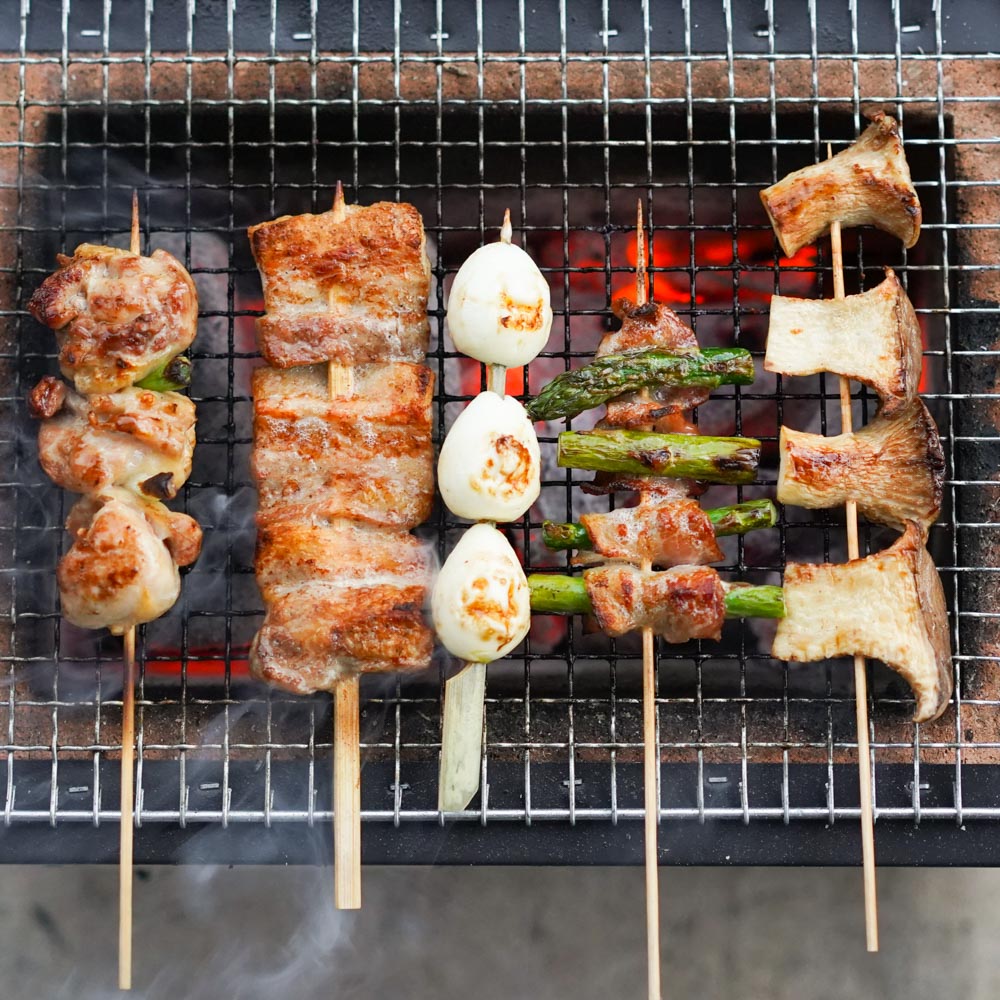The photograph captures an overhead view of a barbeque grill with silver metal mesh over a fire pit, where flames lick upwards from beneath, adding a rich ambiance to the scene. The grill has five wooden skewers with a diversity of foods, showcasing a tantalizing array of culinary delights. From left to right, the first skewer holds chunks of lightly seared chicken. Next, there are larger, more heavily grilled pieces of pork or beef. The third skewer features three small, charred, white eggs, possibly quail eggs. Moving along, the fourth skewer presents a fresh green vegetable that appears to be asparagus, possibly wrapped in bacon. Finally, the fifth skewer rests large, oyster mushrooms that bear a slightly burnt exterior, enhancing their flavor. The wooden skewers themselves show signs of charring, indicating an intense cooking process over vibrant, orange flames. The food items, resting on the crisscrossed black and gray squares of the grill, look incredibly appetizing and well-cooked. This scene is a vivid depiction of a delightful outdoor grilling experience in full swing.